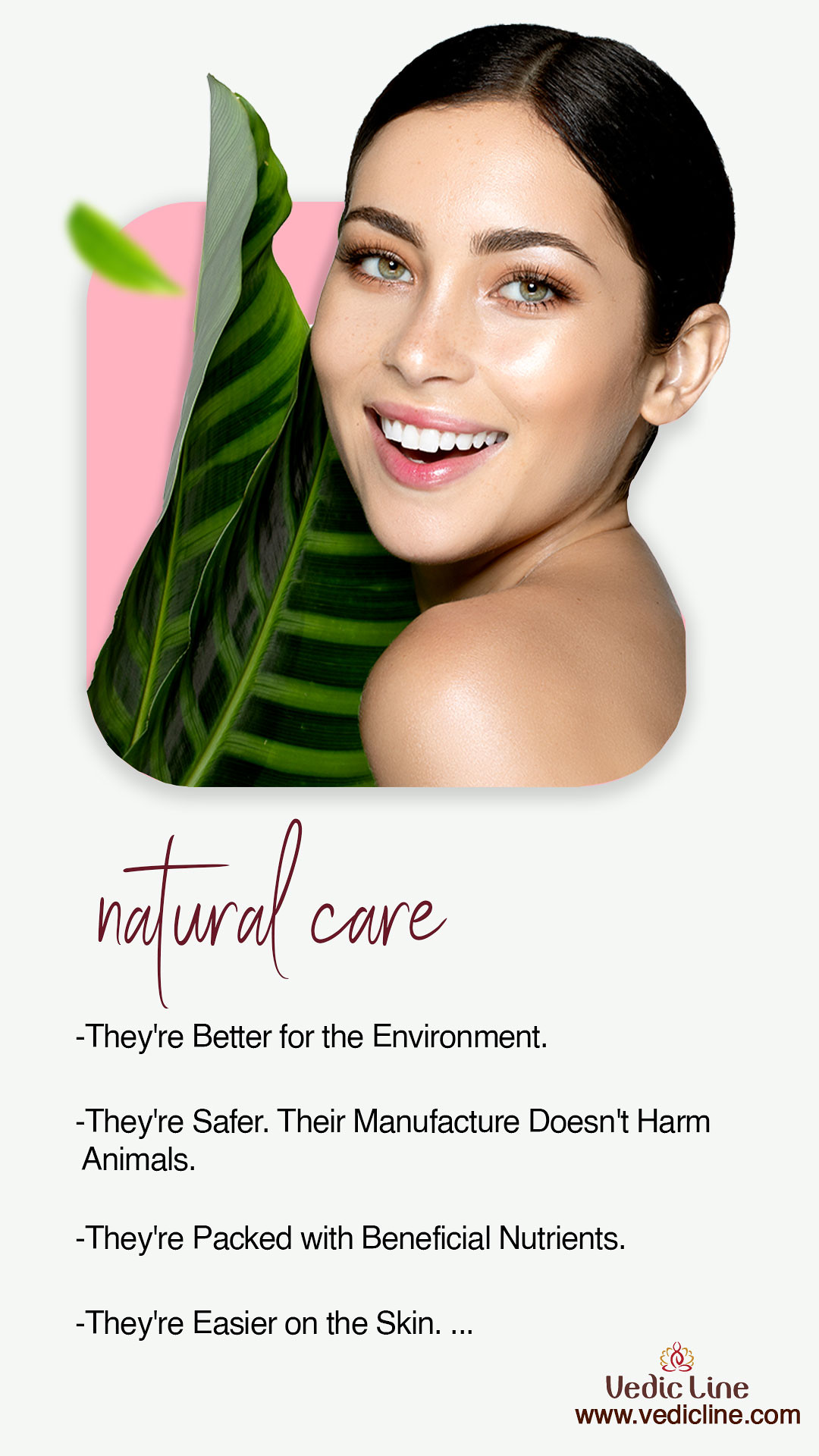The advertisement features a striking image of a woman with dark brown, almost black hair, smiling warmly at the camera. Only her exposed shoulder is visible, suggesting a natural and minimalistic aesthetic. Her skin appears smooth, tan, and glowing, highlighting the effectiveness of the skincare products being advertised. The woman has green eyes and white teeth, set against a pink and white background with giant palm leaves to her left, creating an impression of a tropical, natural environment.

Beneath her image, the text "Natural Care" is prominently displayed, followed by a four-point bulleted list emphasizing the benefits of the products: they are better for the environment, safer, their manufacturing process does not harm animals, they are packed with beneficial nutrients, and they are easier on the skin. In the bottom right corner, the brand name "Vedic Line" is written in brown, alongside the website "www.VedicLine.com." This layout suggests a polished, eco-friendly skincare advertisement promoting the harmonious blend of nature and science.